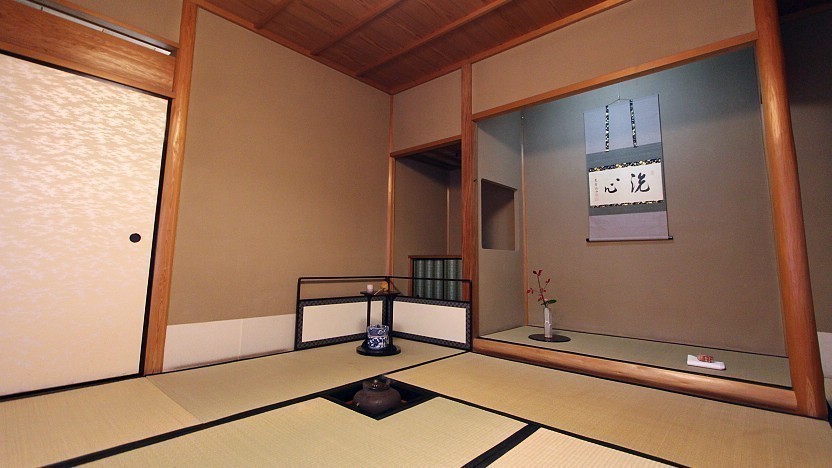The photograph captures an indoor setting suggestive of a traditional Japanese tea room. Central to the image is a blue and white pot or vase, situated on a black plate resting on the floor. Directly beneath, within a recessed black compartment, lies another pot, seemingly made of black stone, suggesting its use for heating tea.

The room features a door on the left side, cream-colored and framed in black wood, with a doorknob placed centrally on the right. Adjacent to the door is a section of brown wall with a light-colored baseboard running horizontally across the middle of the image. This area corners sharply to the right, where it meets another wall fitted with a small, black railing and a blue and white pot resting in front of it.

To the right of this structure, the wall forms two recessed niches. The left recess features brown-colored walls and an undecipherable object, while the adjacent recess contains darker brown walls and a platform holding various items, topped by a wall hanging adorned with Japanese characters and imagery. A compartment on the left recess allows access to another similarly styled open area.

The room’s floor varies in shades of gray and brown, with a prominent recessed area in the middle holding the described pot. A neatly organized component of the room includes an open closet on the right side of the image, which displays a Japanese print calendar and houses a small vase with green sprouting plants and a napkin.

The walls are primarily gray with white highlights along the baseboards, interrupted by brown wood framing. Additional elements include a light fixture above the left door, a pictorial wall hanging featuring black motifs, and a light brown post with a hook, giving the room its distinctive aesthetic.